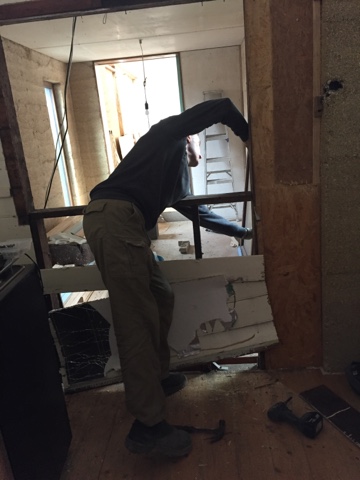In this image, a gentleman is leaning to one side, wearing khaki pants and a green or grayish top, though the poor lighting makes it difficult to discern the exact color. By his feet, there is a hammer, and just to the right, a drill sits on the gray floor. Near his knee, there is some brown insulation, possibly pulled down, adjacent to what appears to be either drywall or wood. He seems to be leaning over a brown wooden frame. To the right side of the frame, brown plywood can be spotted forming part of the wall.

In the background, a white wall partition is visible, with a gray ladder leaning against it. Light filters through what might be a window, or an opening leading to another room with a window. The upper portion of the image showcases a white ceiling, although it is cut off halfway. To the left side, a gray wall with a door opening can be seen, and a wire hangs down from the center left to the bottom left. The floor is made of brown plywood, adding a rustic touch to the scene.